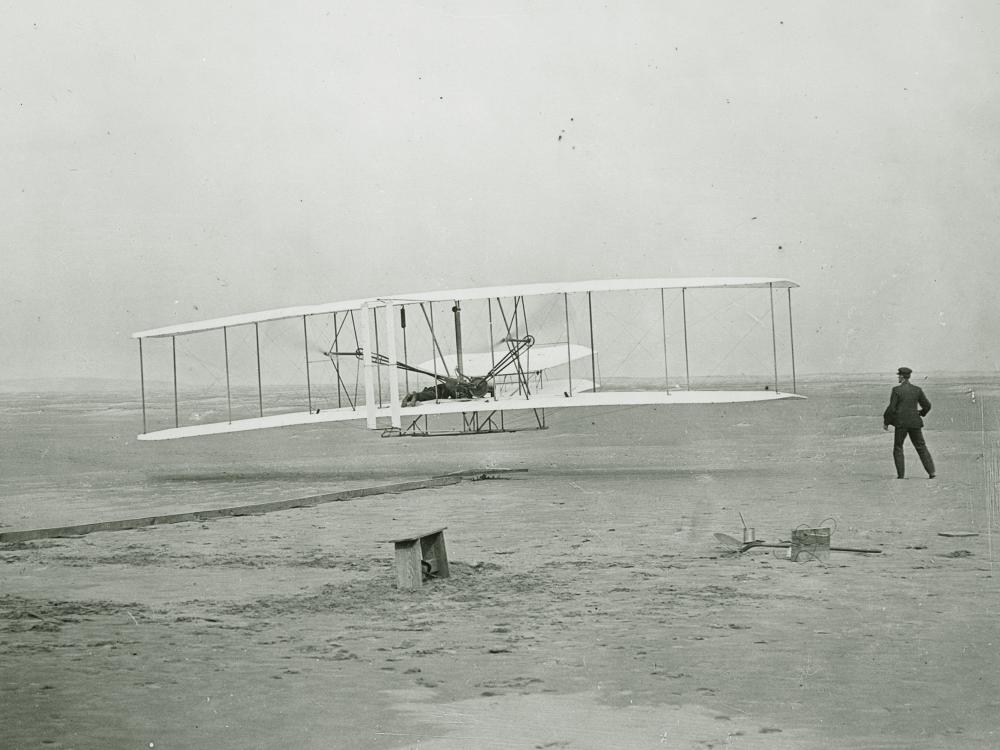This black and white photograph captures a vintage biplane, reminiscent of the early Wright brothers’ models, with its distinctive double-layered horizontal white wings, supported by vertical black struts. The plane, likely an antique from many years ago, features visible mechanical components at its center, which appear to be part of its engine. The aircraft sits on a flat, sandy expanse, possibly a beach, under a gray, clear sky. To the right side of the image, there is a man dressed in a black suit—perhaps a pilot or crew member—standing and observing the aircraft. Additionally, a solitary wooden bench is placed on the sandy ground, adding to the image's deserted and historical atmosphere.